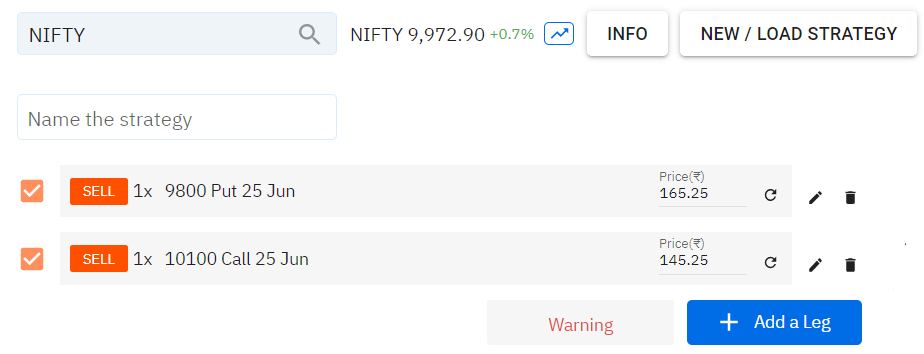The website interface displays a minimalist design with a predominantly white background. At the top, there's a search bar labeled "NIFTY," accompanied by the current index value of "$9,972.90" in bold, next to a green indicator showing a "+0.7%" increase. Below the index information, two clickable tabs labeled "Info" and "New/Load Strategy" are present. 

Beneath the tabs, a box prompts the user to "Name the Strategy," followed by two separate sections outlining trading actions. The first section details "Sell 1 x $9,800 Put, 25 June" priced at "$165.25." The second section specifies "Sell 1 x $10,100 Call, 25 June" priced at "$145.25." This page appears to be part of a stock trading platform where users can execute options trading strategies by selling various stock options.